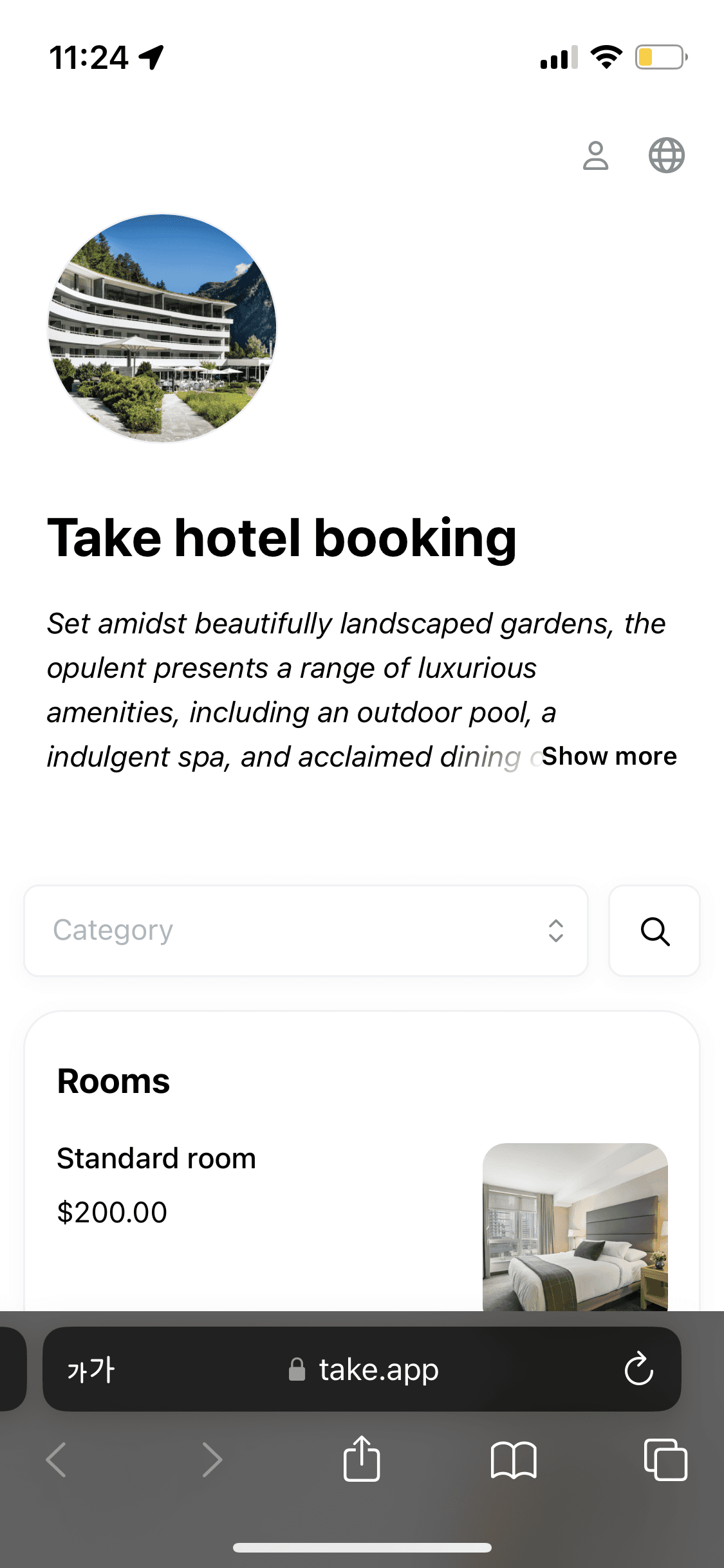Screenshot of a Smartphone Displaying a Hotel Booking Website

The screenshot captures a smartphone displaying a web page from "take.app," as evidenced by the web address bar at the bottom of the screen. The upper part of the display shows typical smartphone icons, including battery percentage, signal strength, and Wi-Fi connectivity, with the current time marked as 11:24 AM. A black location arrow is situated to the right of the time.

In the center of the screen, the mobile website headline reads "Take Hotel Booking" in a bold, dark font. Below the heading is a smaller, lighter-colored font that describes the hotel: "Set amidst beautifully landscaped gardens, the opulent presents a range of luxurious amenities including an outdoor pool, an indulgent spa, and acclaimed dining." There is a "Show More" link for additional information.

Above the textual content is a circular image depicting the hotel. The photo features a several-story, white-colored, flat-roofed building set against a backdrop of a clear blue sky and surrounded by lush green trees.